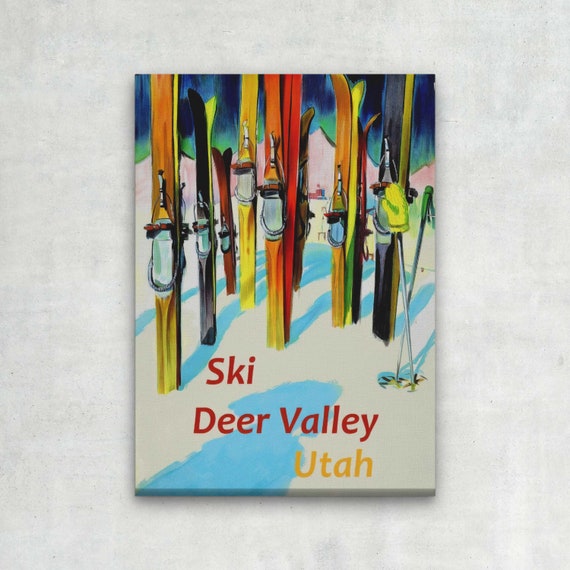The image appears to be a vibrant, vertical canvas art print with a textured ivory and blue background designed to resemble snow. At the bottom of the artwork, bold red text proclaims "Ski Deer Valley," with "Utah" written underneath in yellow. The scene showcases a variety of skis—yellow, orange, red, green, gold, brown, and black—standing upright in the snow, with two ski poles crossing on the right, one topped with a green mitten. There are noticeable blue shadows in the snow, adding to the wintry atmosphere. The background features tall, pink-tinted, snowy mountains and an aurora borealis shimmering above, enhancing the picturesque quality of the painting. The artwork is framed and wrapped like a painter's canvas, giving it a textured, tangible feel, and is displayed against a white and gray stone-like wall.